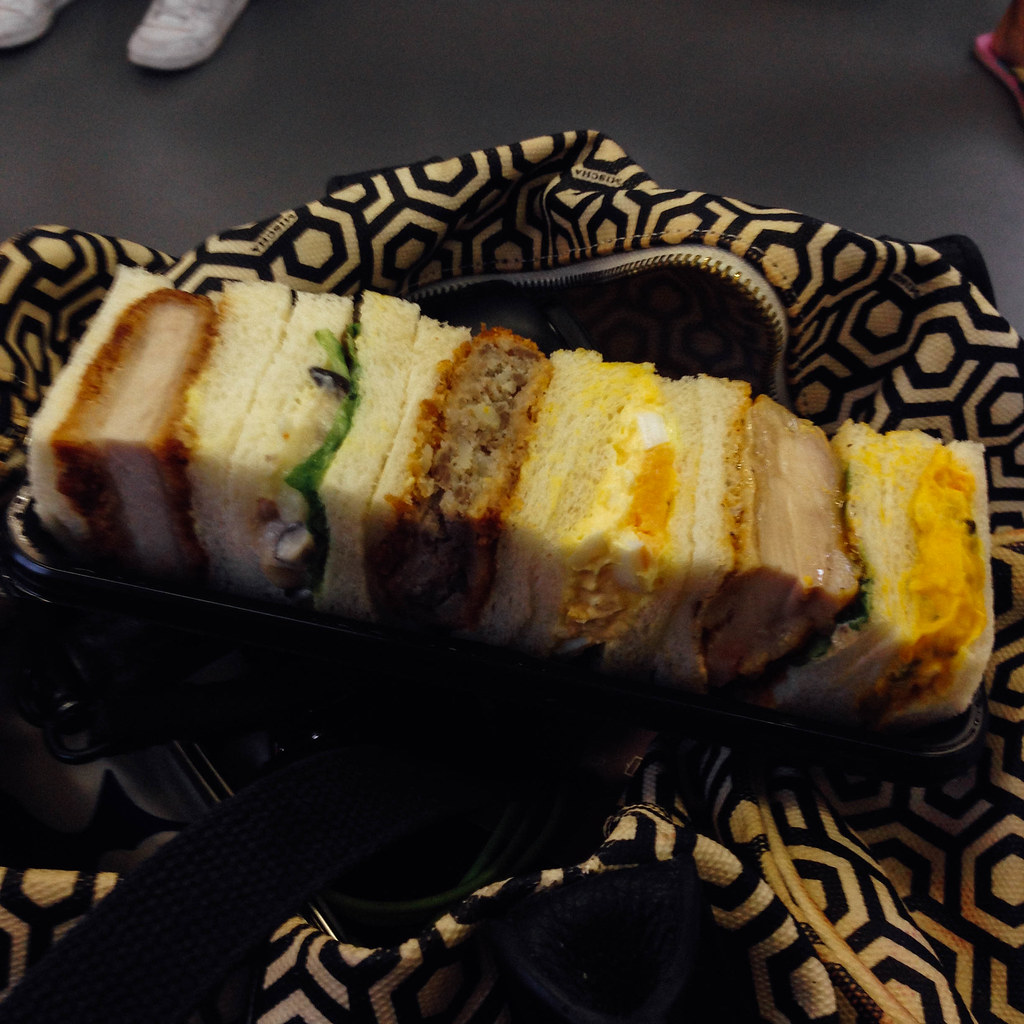This is a square color photograph depicting an assortment of small, square-cut sandwiches arranged tightly together on a black, rectangular tray with rounded corners. The sandwiches, meticulously free of crusts, feature a variety of fillings, including fried chicken, cucumber, chicken salad, meat (possibly chicken fried steak or pork), egg salad, cold cuts, and a mixture of cream cheese with green onion. The tray rests atop a bold-patterned bag, likely a duffel or purse, which is adorned with a prominent honeycomb design in brown and yellow or gold. A zipper with gold-colored teeth is partly visible, indicating the bag is open. In the upper section of the image, the dark floor background is apparent, and part of someone's foot sporting white sneakers, possibly Converse, is visible. The photograph, with slightly out-of-focus details, suggests a casual indoor setting where sandwiches are served as hors d'oeuvres.